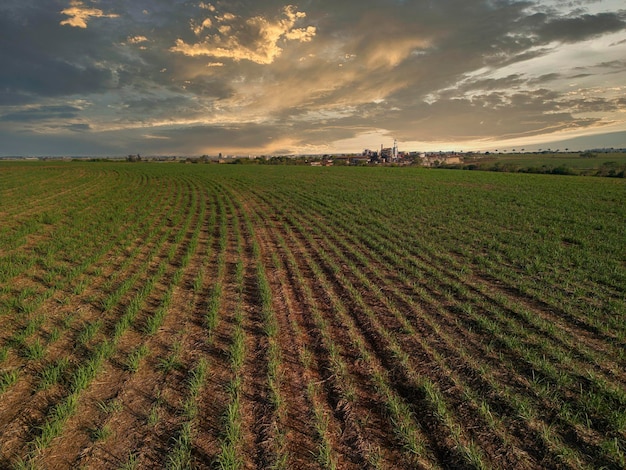This wide-angled color photograph captures an expansive, cultivated farmland stretching across the entire frame. The neatly planted rows of green crops contrast with the brown dirt in between, and the flat landscape enhances the sense of vastness. The sky above is overcast with clouds. The central clouds are illuminated in golden hues, suggesting that the photo was taken either at sunset or sunrise, adding a warm glow to the scene. Hints of blue sky peek through at the top right, while the bottom left showcases gray clouds in the distant horizon. To the right of the image, a small town or cluster of buildings is faintly visible, adding a human element to the otherwise rural setting. The left side remains primarily open farmland. This serene image lacks people, animals, and machinery, emphasizing the tranquility and expanse of the agricultural landscape.